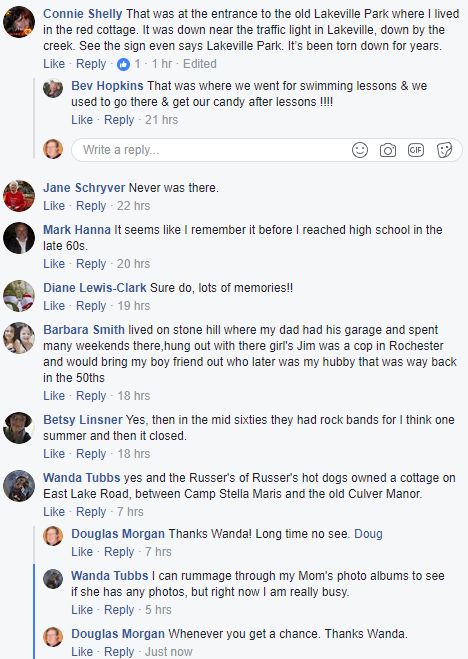The image is a detailed screenshot of a Facebook conversation, showcasing a nostalgic thread about Lakeview Park. The initial post by Connie Shelley reminisces about the entrance to the old Lakeview Park, mentioning her residence in the red cottage near the traffic light by the creek, highlighting that the sign indicating Lakeview Park, torn down for years, is visible. Following her post, Bev Hopkins fondly recalls taking swimming lessons and getting candy there afterward. Jane Shriver adds a brief comment about a location, "Neverville," while Mark Hanna remembers the park from before he reached high school in the late '60s. Diane Lewis-Clark contributes by mentioning the numerous memories she associates with the park. Barbara Smith shares a detailed memory about living on Stonehill and spending weekends at the park, even mentioning a cop named Jim from Rochester who became her husband. Betsy Langsner notes that in the mid-'60s, the park featured rock bands for a summer before it closed. Wanda Tubbs confirms the park's significance, adding that Russer's Russets of Hot Dogs owned a nearby cottage. The thread also includes repeated participation from Wanda Tubbs and Douglas Morgan. The Facebook format distinctly displays profile icons, highlighted names, and reply and like options with timestamps under each comment, creating a vivid community memory quilt centered on the now-absent Lakeview Park.